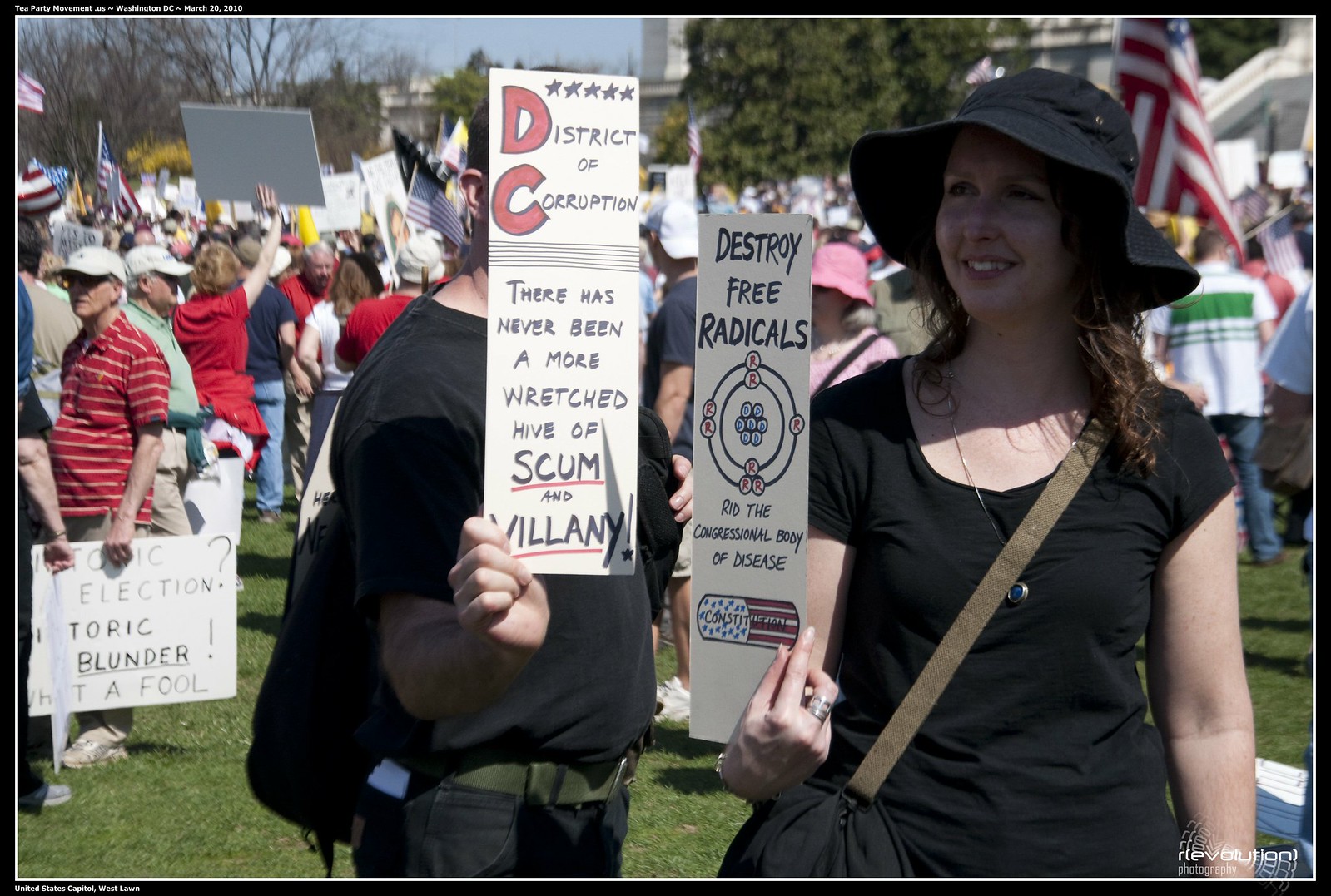In this photograph, a vibrant daytime protest unfolds on a grassy area, highlighted by numerous demonstrators holding homemade signs against a backdrop adorned with several American flags. The focus of the image is a woman positioned prominently in the foreground on the right, dressed in a black shirt and black hat, with a shoulder bag slung across her chest. She brandishes a sign that reads, “Destroy free radicals, rid the congressional body of disease,” accompanied by an illustrative atom featuring Republican icons orbiting a Democrat nucleus, and a band-aid labeled “Constitution.” Standing beside her, a man dressed in black, his face obscured by his sign, carries a poster declaring, “District of Corruption. There has never been a more wretched hive of scum and villainy.” Additionally, to the left, a man in a red and white striped shirt holds a sign stating, “Historic election? Historic blunder! What a fool.” The image is bordered with a black and white frame, emphasizing this captured moment of fervent civic expression.